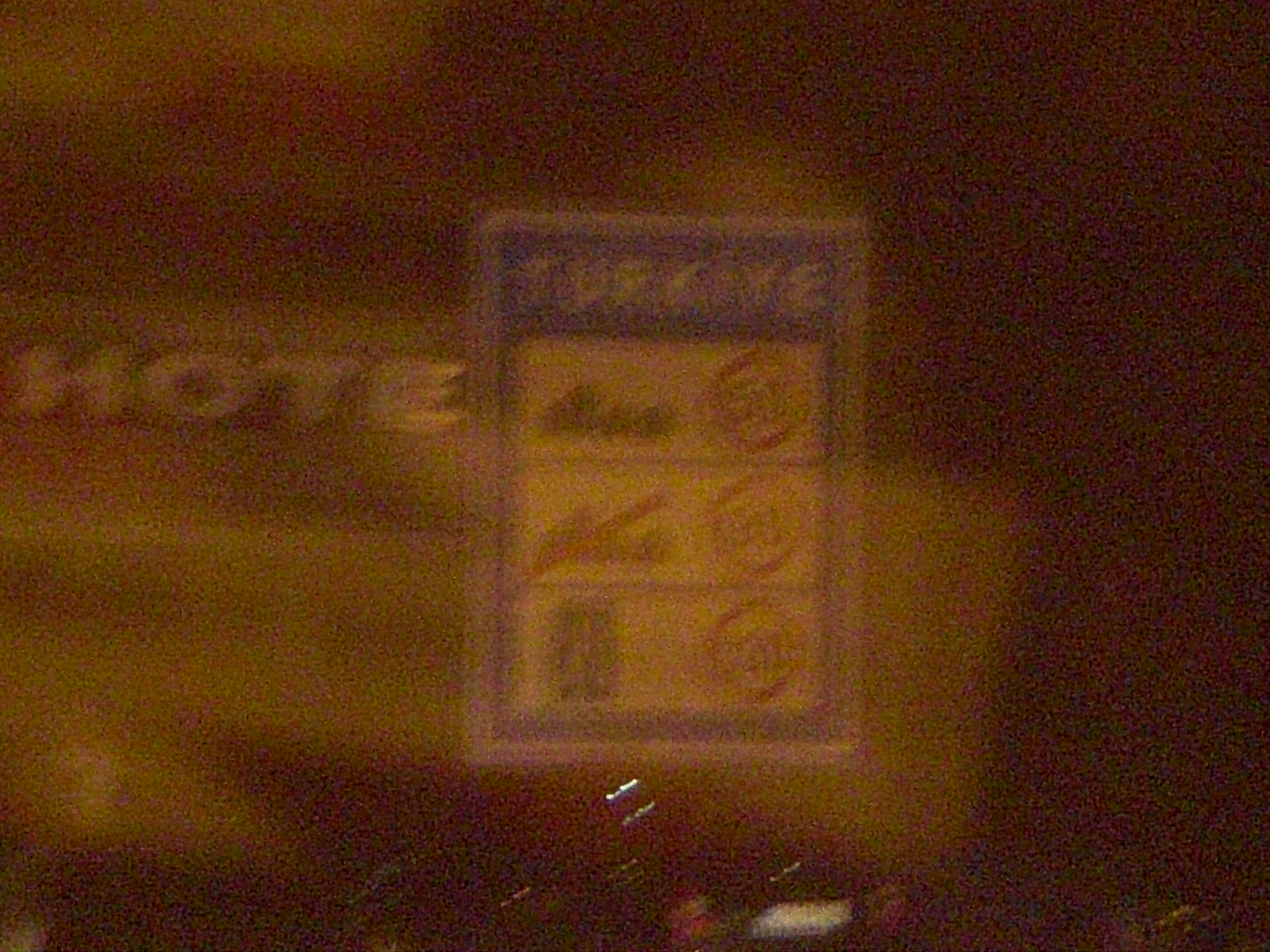In this very blurry nighttime photograph, the poorly visible scene features a blue square road sign broken down into three smaller rectangular signs, each displaying numbers within red circles that might indicate vehicle weight limits or speed limits. The sign prominently features the word "TÜRKİYE" at the top, suggesting a location in Turkey. The image appears to have been taken from inside a moving car, possibly through a window, contributing to the overall blurriness. Adding to the visual confusion, there seems to be a double exposure effect, causing a large, partially obscured "HOTEL" sign in large capital letters to appear in the background. The entire scene is difficult to discern due to its grainy and indistinct nature.